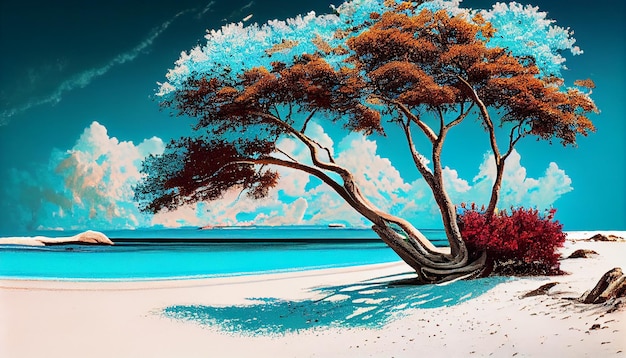This pop art style illustration depicts a serene, white sandy beach contrasted against crystal blue waters that are strikingly still, with no waves in sight. Dominating the scene is a gnarly old tree situated on the beach, characterized by multiple trunks gnarled and knotted together at the base, leaning towards the water. The tree’s foliage is an eclectic mix of bright blue, orange, and rust-colored leaves, with some bunches of turquoise at the top and brownish lower branches. To the right of the tree is a vibrant red bush that adds to the surreal color scheme. The beach also features some scattered rocks. The horizon showcases fluffy white clouds, adding depth to the sky, which darkens toward the left side hinting at an approaching storm. Overall, the vivid, unnatural colors give the scene a striking, dreamlike quality, reminiscent of a colorized photograph or a watercolor painting.